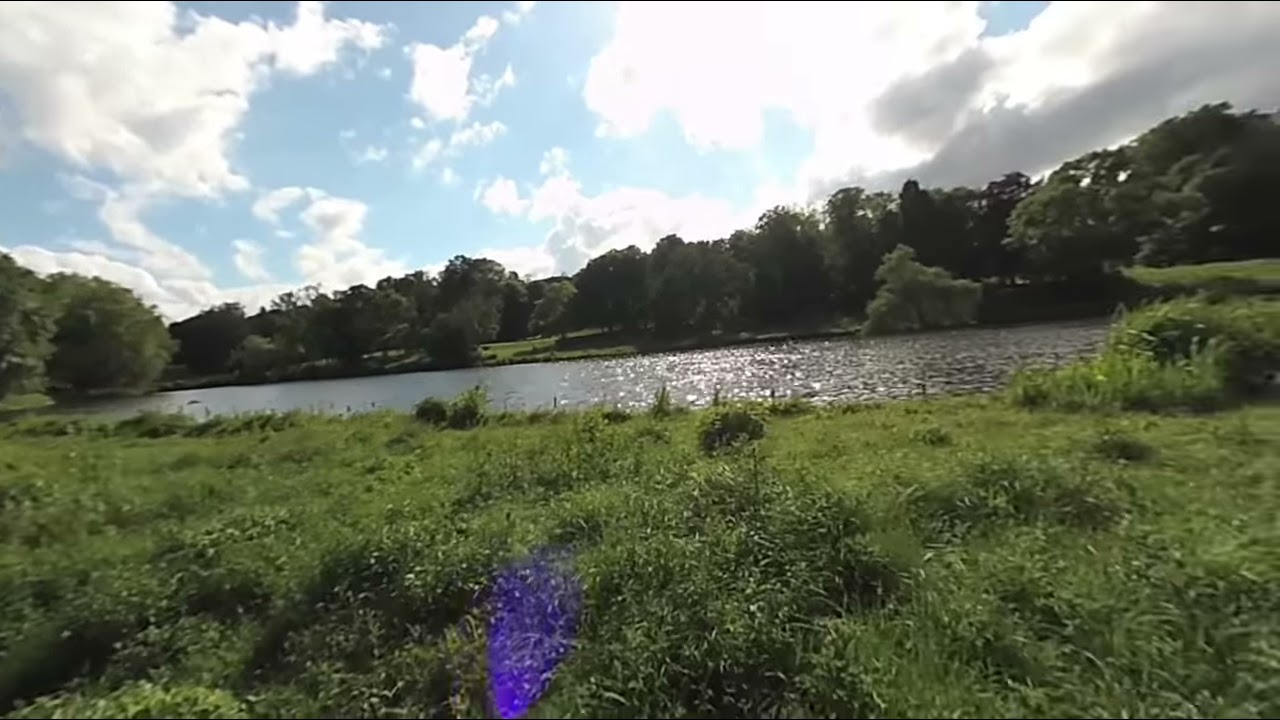The photograph captures a serene landscape, likely taken in the countryside or a secluded park during the day. The sky above is a soft light blue, dotted with various shades of gray and white clouds, through which the sun partially peeks at the top center, casting a diffused light over the scene. The composition of the image, wider than it is tall, resembles the shape of a high-definition TV screen.

Dominating the bottom half of the image is a lush, green carpet of wild grasses and plants leading to the edge of a body of water. This water body could either be a lake or a river, as the image's edges cut off both sides, preventing a definitive identification. The water itself is tinged brown and glistens under the sun's reflection.

The far shore of the water features more green grass and a dense cluster of trees, contributing to the sense of isolation. Notably, there are no signs of human habitation or presence anywhere in the photograph, reinforcing its tranquil and untouched nature. 

In the lower part of the image, a purple splotch appears, likely a lens flare or camera distortion, while a similar blue spot can be seen in the lower center left, possibly indicating slight diffraction of light. Additionally, the position of some grasses suggests a gentle breeze might be blowing across the landscape. Overall, the photograph encapsulates the peaceful beauty of a natural, unspoiled environment.